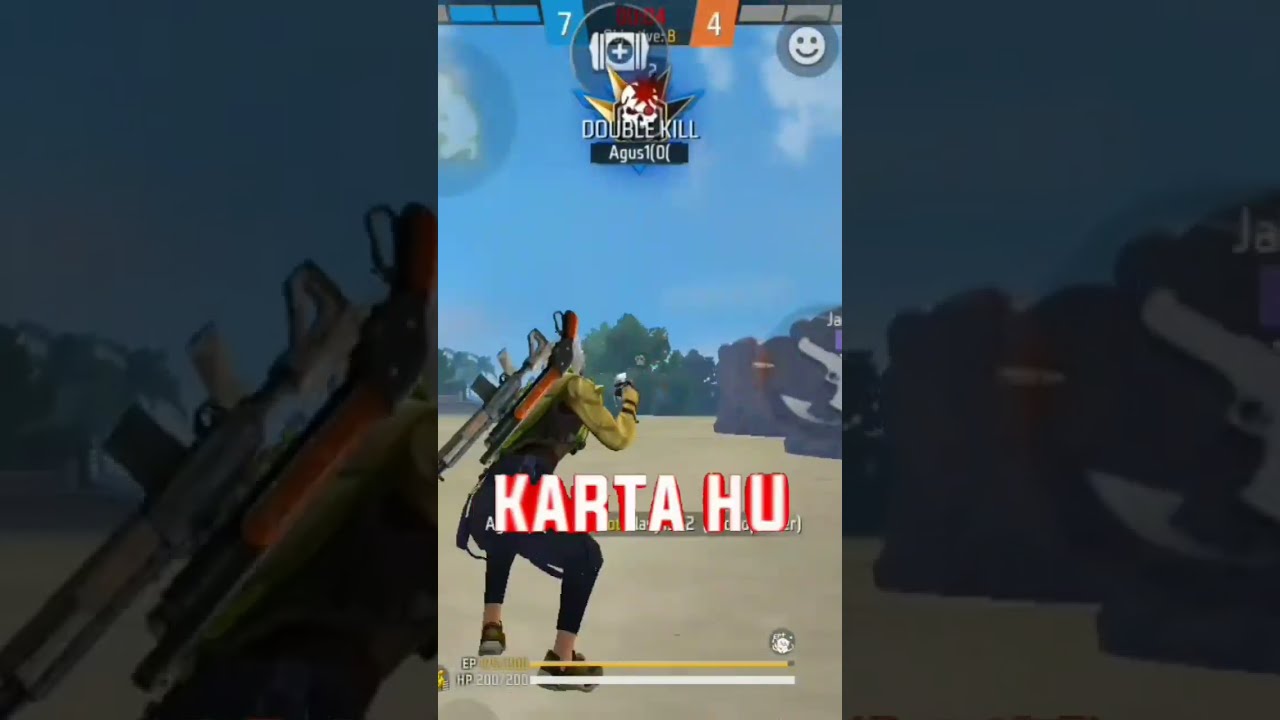The screenshot captures a third-person shooter video game in a bright, outdoor setting beneath a clear blue sky. The scene is divided into three sections: the left and right thirds are dimmed, zoomed-in portions flanking the more vibrant center third. In the foreground, a character squats, facing away from the viewer, equipped with two shotguns attached downward on their back. Dressed in black pants and a black long-sleeved shirt with yellow sleeves, the character’s gender remains undiscernible. The terrain is light-colored sand, and some brown structures and stone archways are visible on the right, with green trees seen in the distance.

Text overlays the image, indicating game-related information. The top displays "Double Kill A-G-U-S one (0)," alongside a skull with a spike through it and a star with four points, surrounded by blood splatter. Below this, a scoreboard shows the blue team leading with seven points on the left versus the orange team’s four points on the right. Central to the image is the text "Carta Who" (K-A-R-T-A space H-U), accompanied by a happy face icon within a circle. The screenshot suggests an intense, yet graphically simplistic, battle royale gameplay environment.